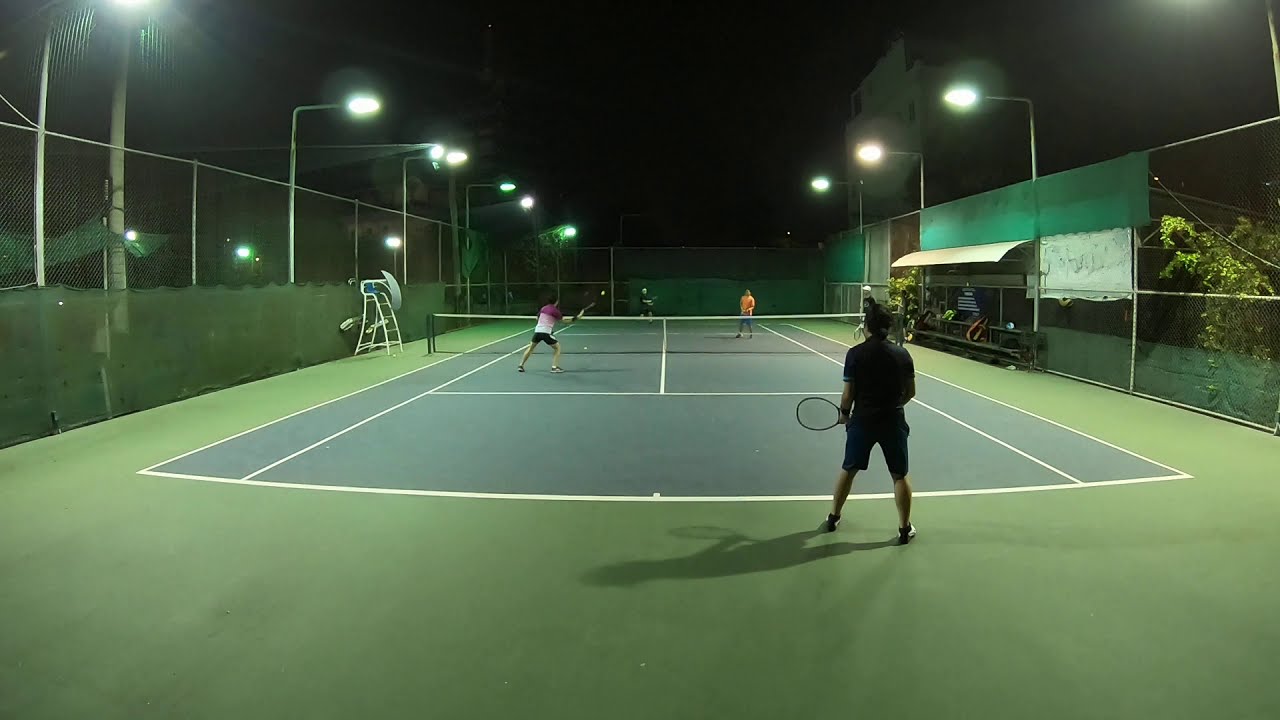This is a horizontally aligned rectangular photo taken at nighttime of a well-lit tennis court surrounded by a tall metal fence. The court, illuminated by multiple overhead lamps that are high in the air, shows a playing surface with a distinct color scheme: light green around the play area with dark green or gray in the center, accented by white boundaries. The background sky is solid black, indicating it is nighttime. 

On the court, there is a doubles game in progress with four players visible. Closest to the camera and standing in the middle, ready for action, is a man wearing dark blue shorts and a black shirt with short black hair. To the left and diagonally near the net, another player is seen wearing black shorts and a shirt with purple and white stripes, appearing to have just hit the ball. On the opposite side of the net, the player closest to it is visible wearing an orange shirt, while the fourth player is too distant to clearly make out. The court also exhibits various green undertones, including green banners or tarp along the left side and the background, and green reflections from the lights. Off to the right is a bench with an overhang, also covered by green tarp, and there are some plants visible nearby.